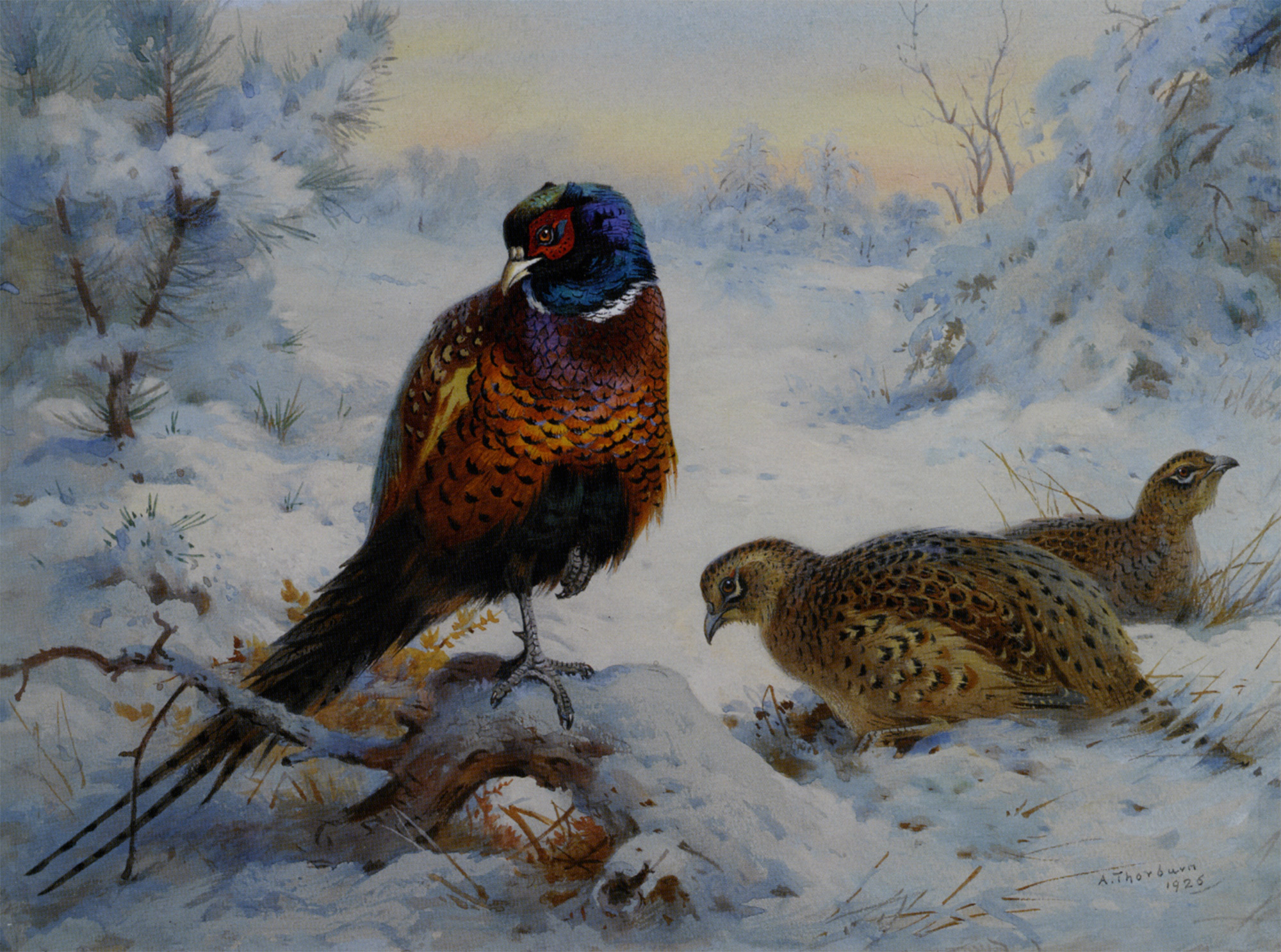In this beautifully rendered painting from 1925 by A. Thornburn, an idyllic winter scene unfolds in a quiet snow-covered forest. The trees, heavily blanketed with fluffy white snow, frame the composition on both the left and right. In the background, another row of snow-laden trees stretches towards a serene horizon, where the sky transitions softly from a warm orange hue to a pinkish off-white, suggesting either dawn or dusk.

The focal point of the painting is three birds nestled in the foreground against the pristine white snow. The most striking bird, positioned on the left, is an adult pheasant perched delicately on a large hunk of wood, possibly a tree stump or branch. This pheasant is resplendent with an iridescent blue head, a white ring around its neck, and a long, elegant tail. Its feathers exhibit a beautiful blend of black, blue, golden brown, and orange hues, and it stands with one foot tucked into its plumage.

Next to the vibrant pheasant are two more birds of the same species, likely younger pheasants or quails, with light brown feathers accented by darker spots, blending harmoniously with the snowy environment. All three birds exude an air of calm, nestled cosily in the tranquil winter landscape.

This artwork captures the delicate stillness of a snowy forest, bathed in the soft glow of either early morning or late afternoon light, presenting a peaceful and detailed study of nature's beauty.